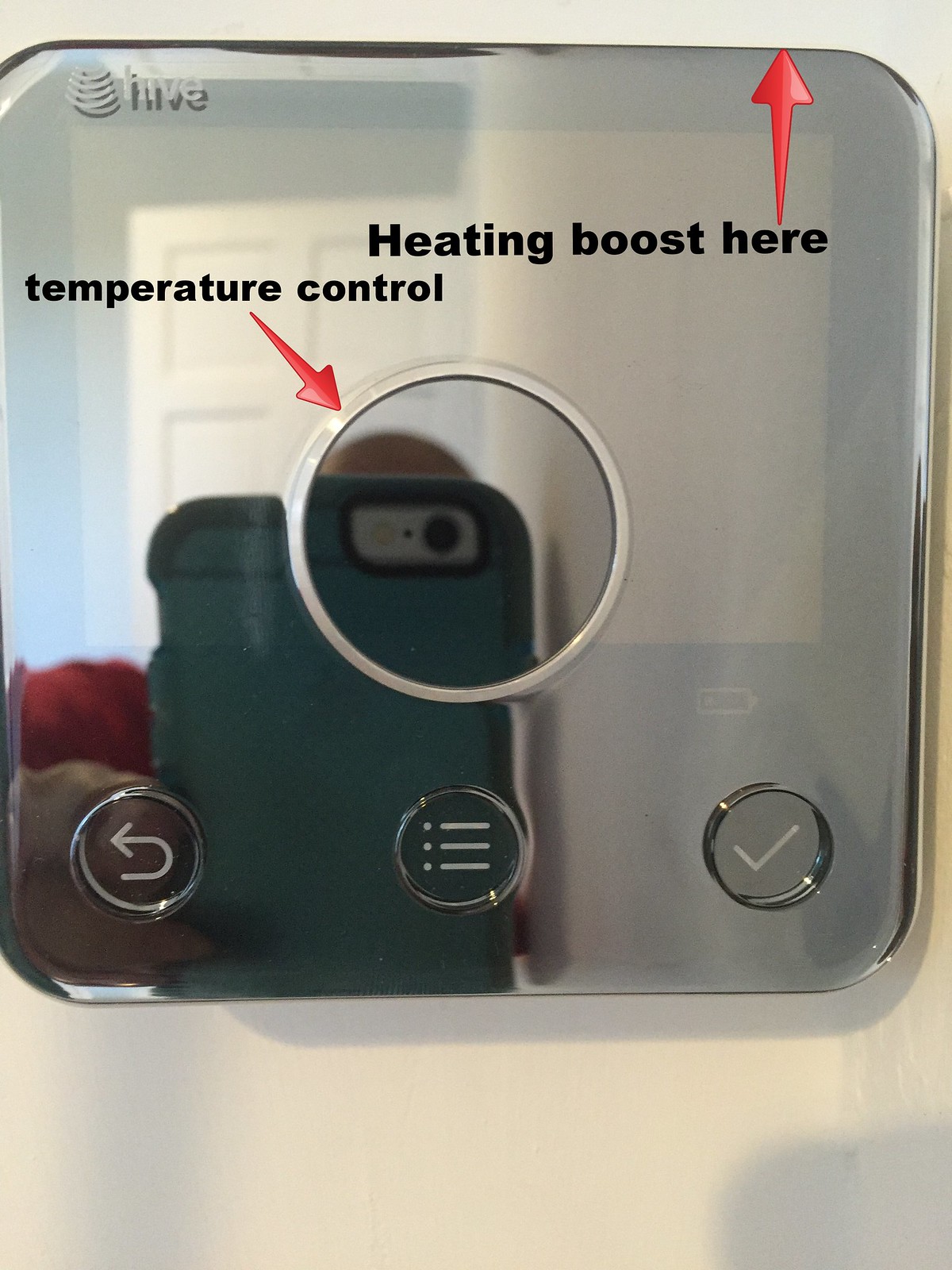This image features a sleek, mirrored surface mounted on an otherwise plain white wall, showcasing a highly polished, silver-colored finish. In the upper left-hand corner, the word "HIVE" is emblazoned in black, accompanied by a small, semi-circular, multi-segment icon, providing a subtle yet noticeable branding element.

On the upper right-hand corner, bold black text reads "HEATING BOOST HERE," with a red arrow directing attention to it, highlighting a specific function. Centrally located on the mirrored surface is a metallic silver ring, also accompanied by a red arrow labeled "TEMPERATURE CONTROL," indicating its primary function.

In the bottom left corner, a U-shaped arrow symbol, resembling an undo button, adds functionality to the interface. The bottom middle of the mirror features a "menu" icon with three dots above three horizontal lines. Finally, in the bottom right corner, a checkmark button is visible, likely serving as a confirmation tool.

Reflected in the surface, a white door can be seen in the background, along with a person holding a phone in a green case, partially obscuring their bald head. The person is wearing a red t-shirt, making the reflection vivid and detailed.